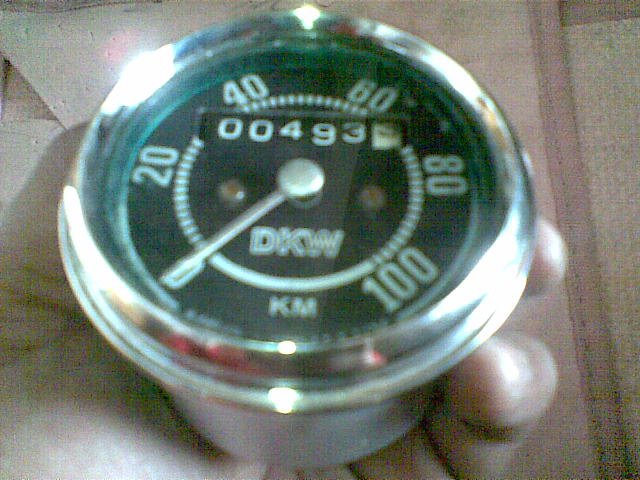In this image, a speedometer is being held by someone whose hands appear to be male, based on their size and appearance. The speedometer itself has a metallic silver casing, with both the bottom and the round top portion shining in silver. The face of the speedometer is predominantly black, with white markings and numbers that clearly stand out. 

Starting from zero and moving clockwise, the numbers increase in increments of 20, reaching 100. The current needle position is at zero. Within the central part of the speedometer, the numbers "00493" are displayed, likely indicating cumulative distance traveled. Directly beneath these numbers are the letters "ZKW," and just below that, under a small horizontal line, is the abbreviation "KM," denoting that the measurements are in kilometers.

The person's hands holding the speedometer rest on what appears to be a wooden table, with a beige cloth partially visible around the edges, adding a touch of warmth and texture to the scene.